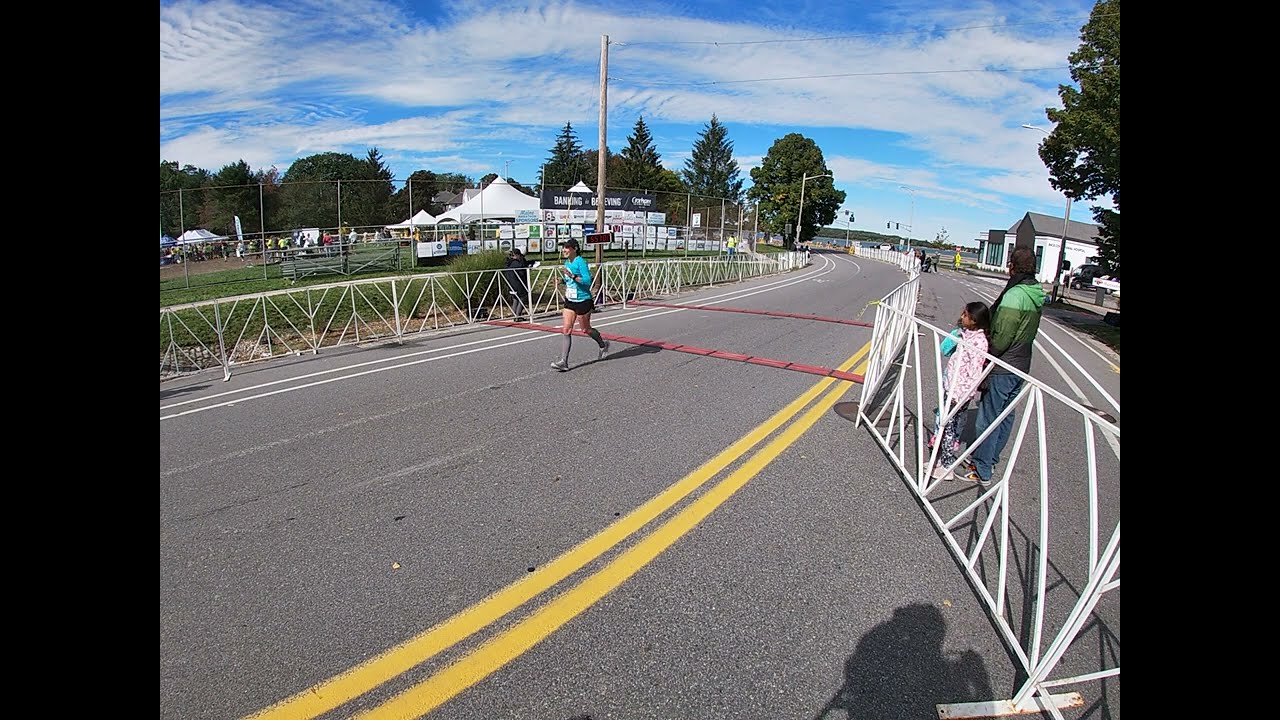The image captures a scene of a blocked-off road, likely for a marathon or race event. The road starts from the lower left corner and curves slightly to the left, extending towards the upper right. The middle of the road features a temporary white barrier fence with diagonal bars, standing approximately three feet high and running along the double yellow lines. On the right side of the road, two individuals appear to be either setting up the fence or leaning against it. The first person is an adult wearing a multi-colored green jacket with a dark and light green contrast, paired with blue loose pants. Next to them is a younger person, wearing a pink jacket, black and white leggings with a floral pattern, and pink shoes.

On the left side of the road, a young woman is running towards the camera, dressed in a teal T-shirt, black shorts, gray socks, and gray shoes. Her stride and attire suggest she is a participant in the race. The road also features white railings extending along its edges and two red strips across it, possibly marking a start or finish line.

The background includes a grassy field to the left, another fence line demarcating the road's edge, pop-up tents, and several white pavilions, adding to the event atmosphere. The sky above is mostly blue with scattered wispy clouds. Additionally, there are telephone poles with lights and some trees visible in the distance, indicating the location is a mix of urban and natural settings.